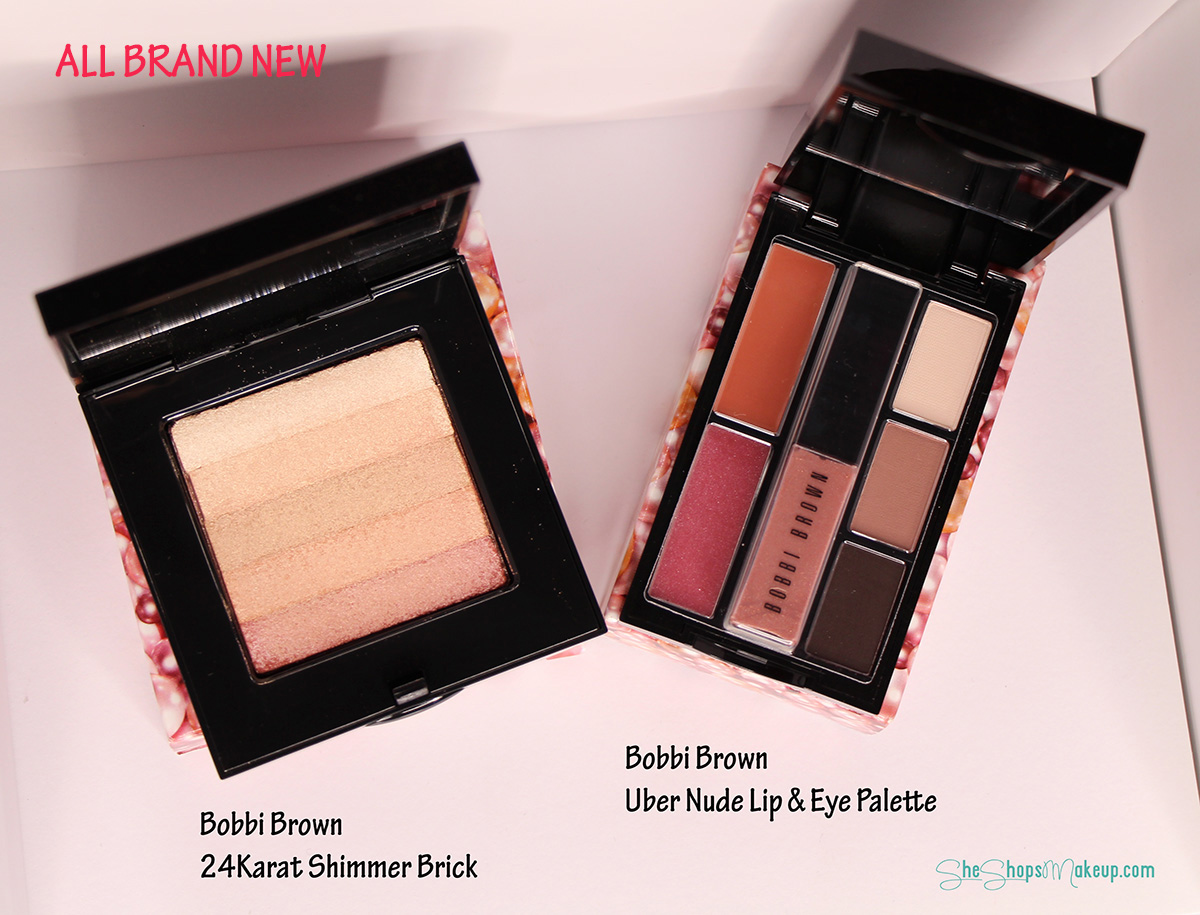The advertisement image from SheShopsMakeup.com features two open makeup palettes displayed prominently against a decorative background with florally pink, peach, and white patterns. Both palettes are in sleek black containers and showcase a stunning array of colors. At the top of the image, the phrase "All Brand New" is written in bold dark pink lettering. 

On the left side, the Bobbi Brown 24K Shimmer Brick is highlighted, featuring a blended spectrum of shades within a single square; the colors transition smoothly from a very light hue to gradually darker tones. On the right side, the Bobbi Brown Uber Nude Lip and Eye Palette is displayed, consisting of seven distinct shades, each housed in its own compartment. These shades range from tan and beige to brownish, reddish, and mocha colors. 

The palettes, likely set on a table or within a display case, are photographed from above, providing a clear view of the makeup's vibrant hues. This detailed advertisement could be seen in a store, an online shop like Amazon, or within a beauty magazine.